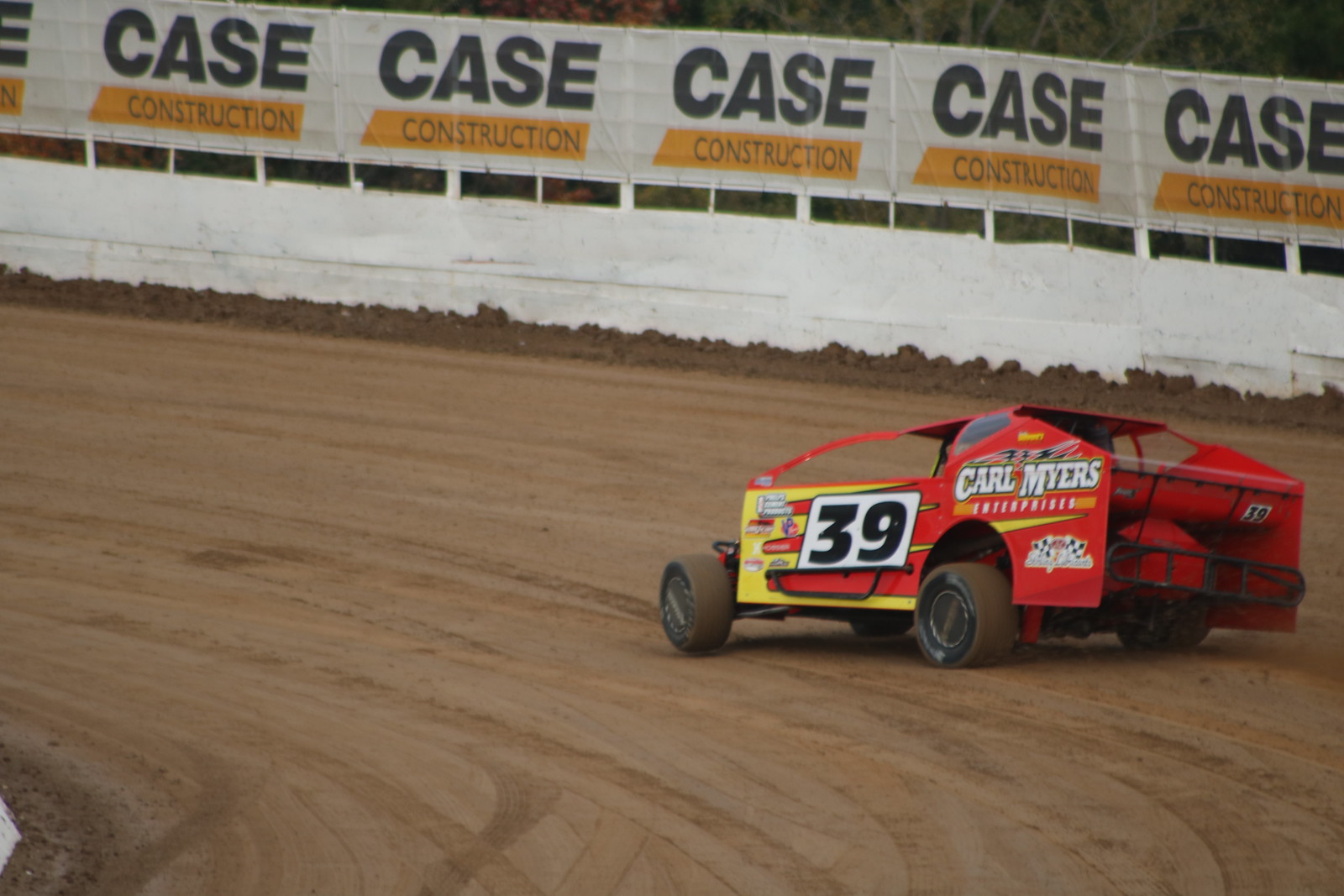The image captures a vibrant red and yellow race car with small, stout wheels tearing through a dirt track in a counterclockwise direction. The car, viewed from the left side, prominently displays the name "Carl Myers" in bold white letters on the back panel and features the number "39" in black within a white box on the door. The track, muddied with visible tire tracks, is bordered by a white concrete fence. Above the fence, a sponsor banner runs across the entire wall, showcasing "CASE CONSTRUCTION" in bold black letters with "CONSTRUCTION" set against a yellow background. This color photo or video freeze-frame, in landscape orientation, offers a detailed and realistic representation of the race setting, complete with surrounding greenery in the upper right corner.